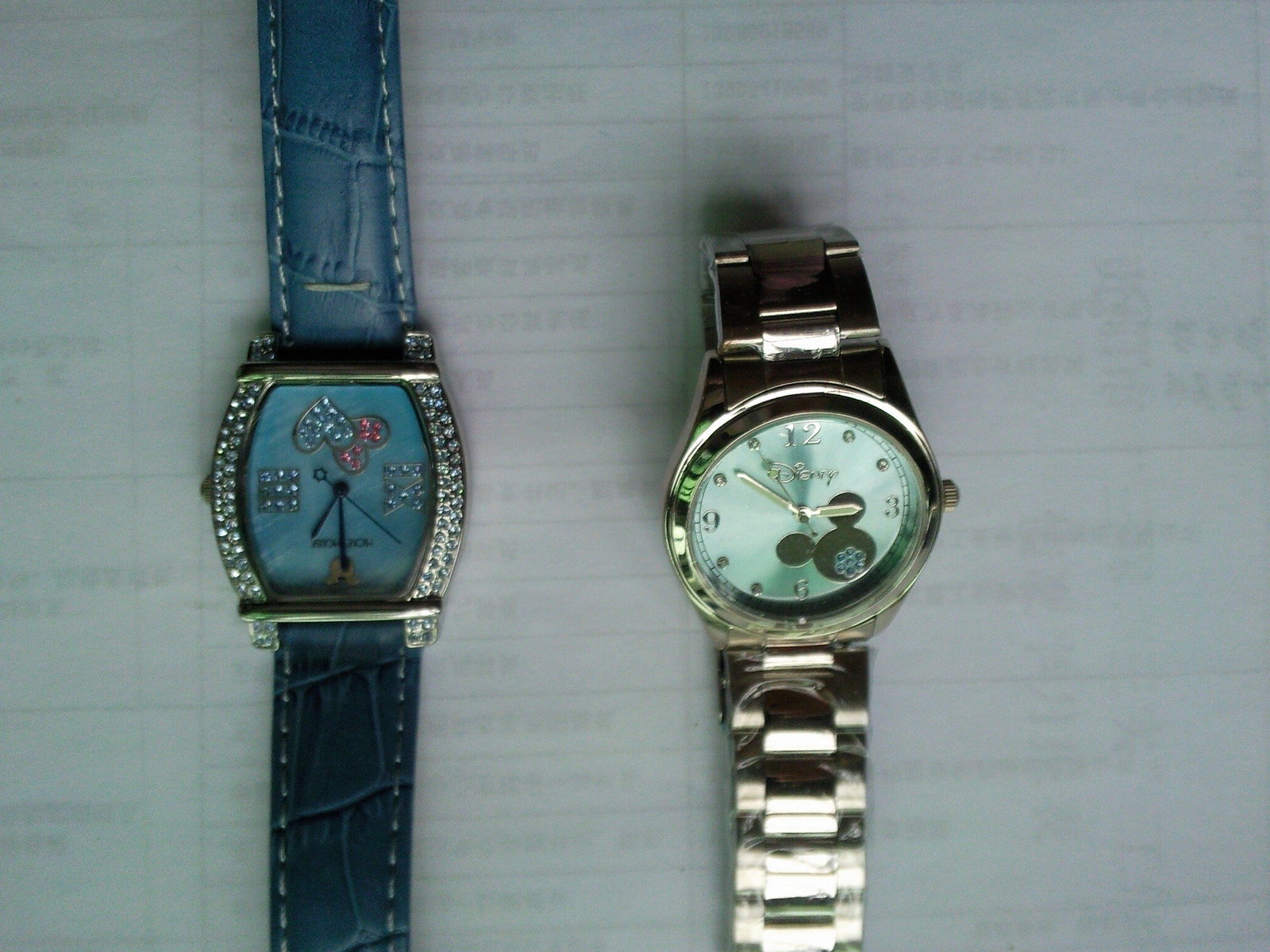This is a vibrant color photograph showcasing two distinct wristwatches placed on a piece of white paper. Slightly discernible text appears to bleed through the paper, though it remains unreadable. 

On the left, an elegant wristwatch features a blue leather crocodile-style strap and is positioned upside down. Its face dazzles with an iridescent blue hue, encircled by shimmering rhinestones. The watch face itself embellishes further with two squares of rhinestones, a rhinestone silver heart, and a rhinestone red heart. A gold Mickey Mouse head marks the 12 o’clock position, adding a playful yet refined touch to the design.

To the right, the second wristwatch boasts a gold chain-link strap and a contrasting light silvery-green face. This watch has a minimalist design, displaying only the 12, 3, 6, and 9 numerals. Near the 4 and 5 o’clock positions, a subtle Mickey Mouse head is nestled, coordinating with the watch’s gold hands. The word "Disney" is elegantly inscribed beneath the 12 in gold lettering, completing the sophisticated look.